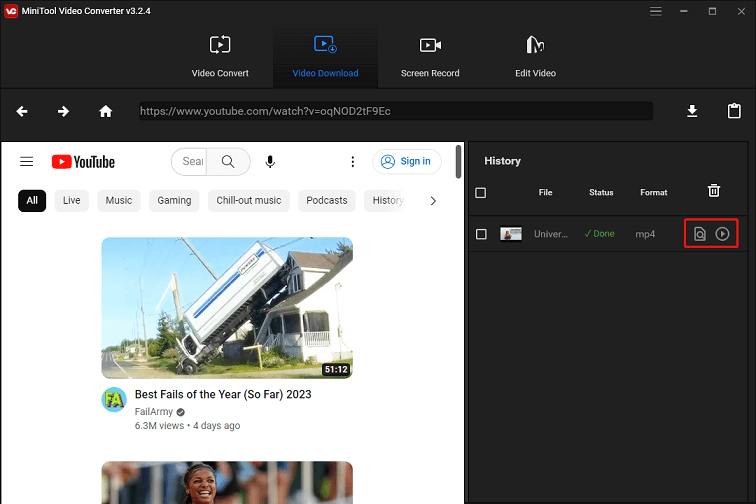Inside the MiniTool Video Converter (Version 3.2.4) program, the computer screen primarily displays a black background. In the top left-hand corner, there is a small red square with the letters "VC" in white, indicating the program's logo. Next to the logo, the program name and version are specified in white text.

At the top center of the application's interface, there are four selectable options: "Video Convert" (highlighted in white), "Video Download" (highlighted in blue, indicating it's the active option), "Screen Record" (highlighted in white), and "Edit Video" (highlighted in white, each with its respective icon).

Beneath these options, there is a navigation bar that includes a left arrow, a right arrow, a home button, and a web address reading "https://www.youtube.com/watch" followed by some letters, indicating the URL of the video currently being downloaded for potential editing. On the far left of this bar, there is a clipboard icon representing tasks. On the far right, there are two tabs: "History" and another checkbox.

Under the "History" tab, there are several columns labeled "File," "Status," "Format," and accompanied by a trash can icon for deletion. Below these columns, there is a label that partially reads "UNIVER" and the status "Done" in green with a checkmark. The format is specified as "MP4," along with two small icons within a red rectangle, showing a page with a magnifying glass and a radial button, presumably for activating the task.

A secondary window has popped up in front of the black screen, likely the YouTube interface. This window features a search bar with a microphone icon, a sign-in option on the top right, and various tabs such as "All," "Live," "Music," "Gaming," "Chill Out," "Music," and "Podcasts." The video currently being viewed is titled "Best Fails of the Year So Far in 2023" from FailArmy.